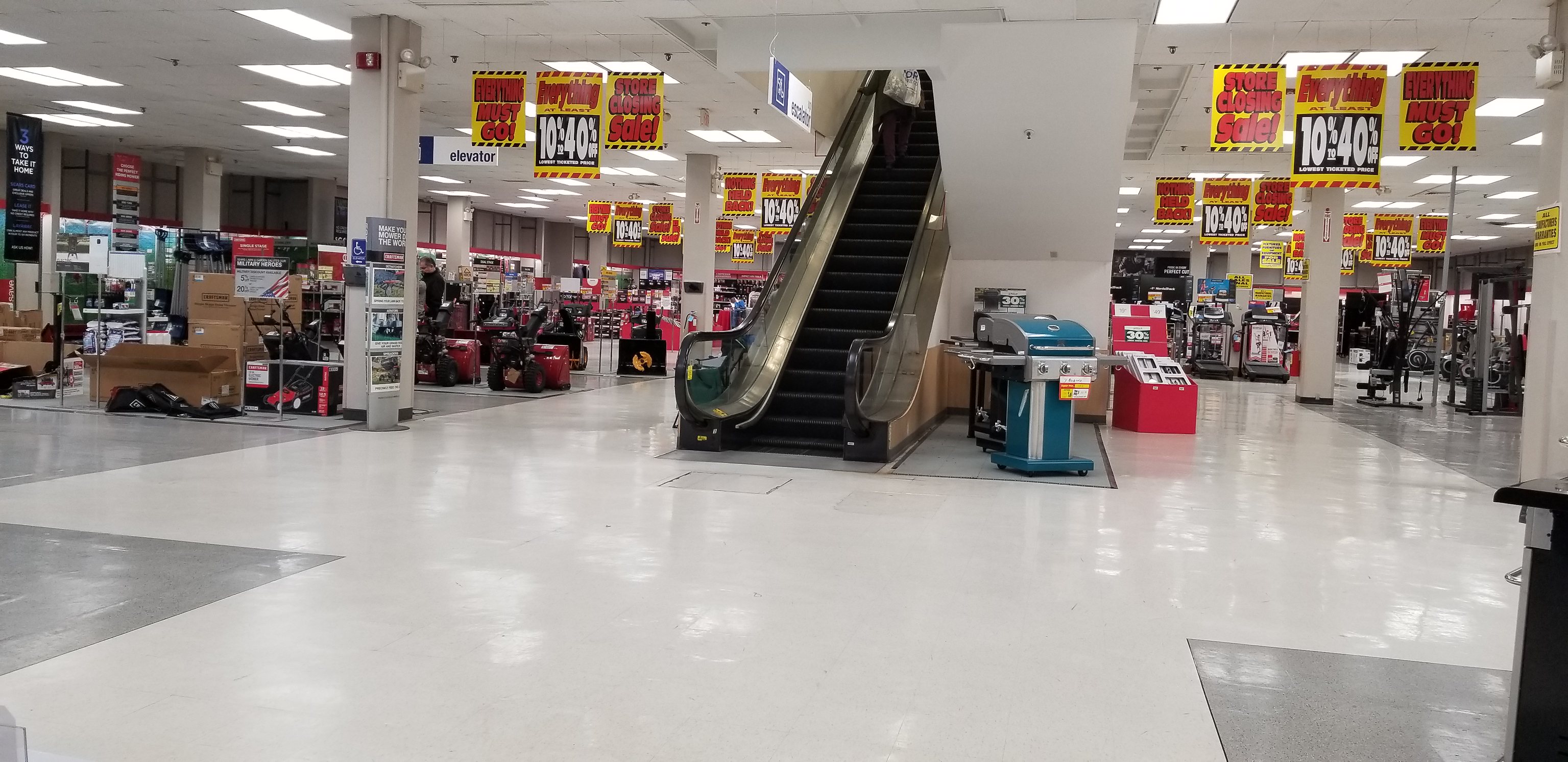In this busy department store scene, a spacious floor is meticulously tiled with a pattern of white tiles bordered by gray ones, creating a clean and organized look. The store's interior features light gray walls and ceilings, which are outfitted with a multitude of ceiling lights, ensuring a bright and welcoming atmosphere. Centrally located is a black and silver escalator, offering easy access to different store levels. Nearby, a conspicuous blue machine stands, although its purpose is not immediately clear. Adjacent to it, a vibrant red rack is filled with various newspapers and magazines. Surrounding these elements, numerous sales signs are prominently displayed, advertising discounts ranging from 10% to 40% off. The store's offerings are diverse, with clothing items prominently featured, as well as a section on the left showcasing various furniture items and luggage, reflecting the department store's extensive and varied inventory.